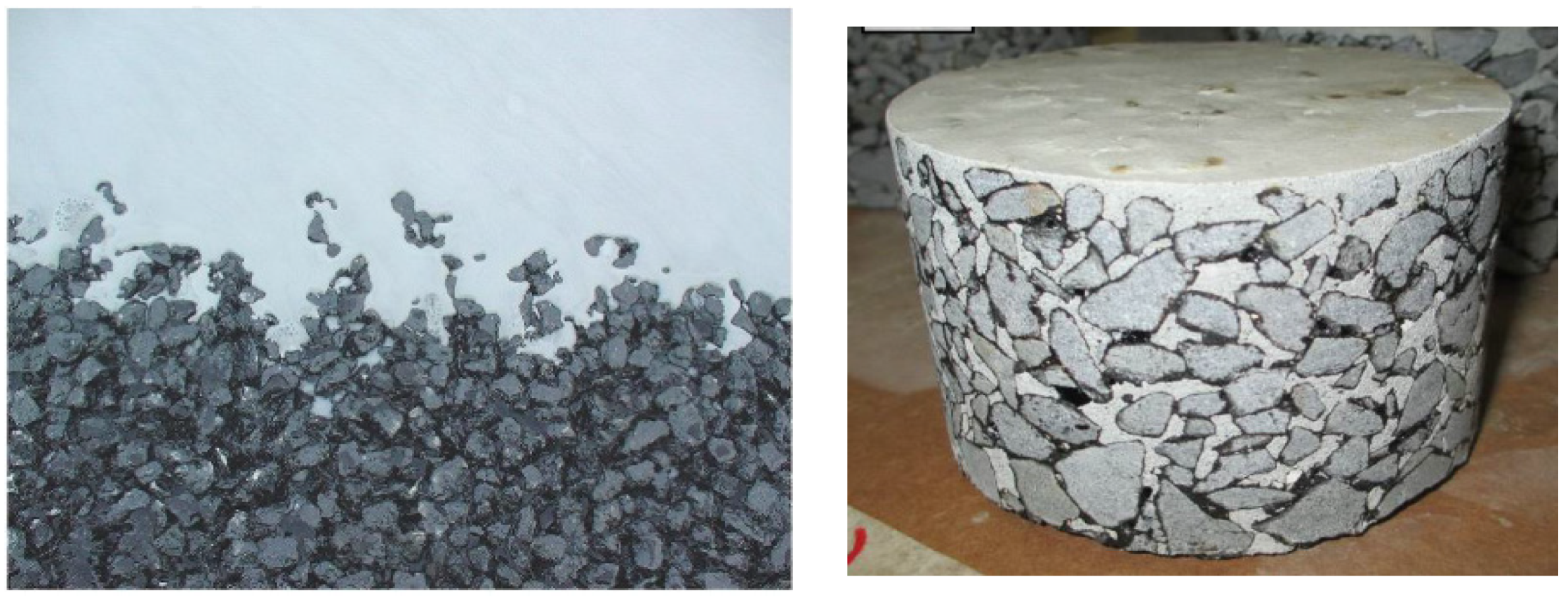The image consists of two side-by-side photographs. The left photograph displays a cluster of irregular, dark gray to almost black rocks or pebbles densely packed at the bottom. Above this heavy aggregation, a few scattered rocks ascend into a light blue background, resembling fragmented asphalt or pavement pieces. The top portion of the rocks appears to be lightly dusted with white, possibly snow. The right photograph features a cylindrical structure with a smooth, white top resembling the icing on a cake. The cylinder is composed of a dense material, possibly concrete, with similar dark gray and black rocks embedded into its surface, resembling marshmallows in a rocky road dessert. The cylinder sits on a light-colored, flat pavement, making the entire structure appear as a meticulously crafted white and gray circular form with a textured rocky surface.